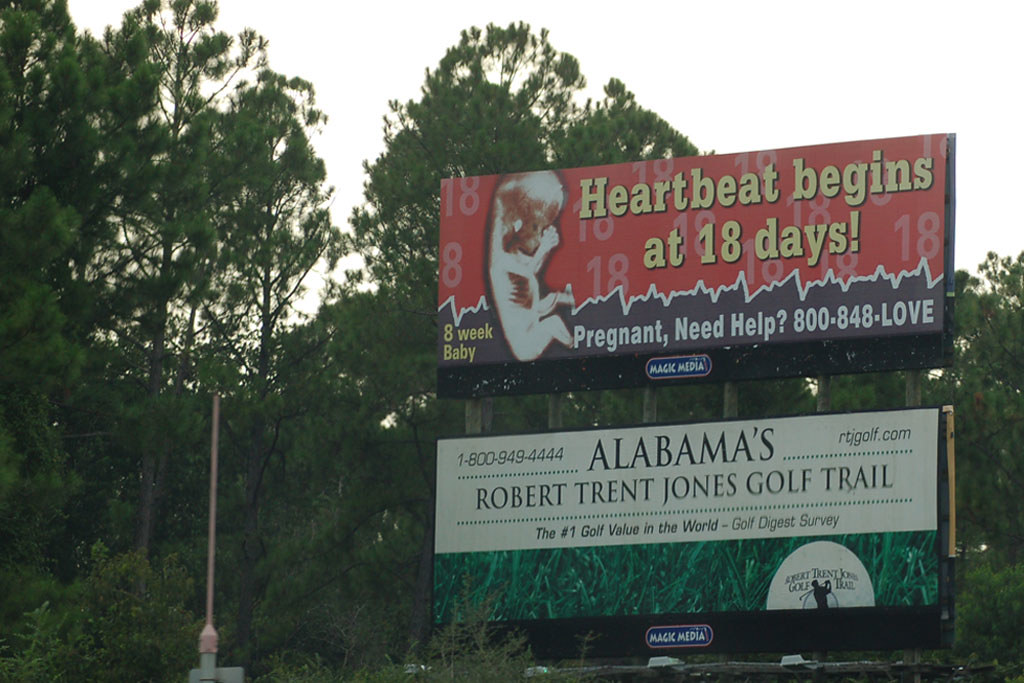This image captures two juxtaposed billboards located off a major highway, likely an interstate, surrounded by tall trees. The upper billboard features a pro-life message with a large, striking image of a fetus. Bold yellow letters state, "Heartbeat begins at 18 days," alongside the text "8 week baby." It includes a helpline number, "800-848-LOVE," for those seeking assistance during pregnancy.

Below it, a contrasting advertisement promotes "Alabama's Robert Trent Jones Golf Trail." This billboard advertises the golf trail as "the number one golf value in the world," featuring an 800 number (800-949-4444) and the website rtjgolf.com. The graphic includes an icon depicting a man mid-swing with a golf club, subtly integrated into the design.